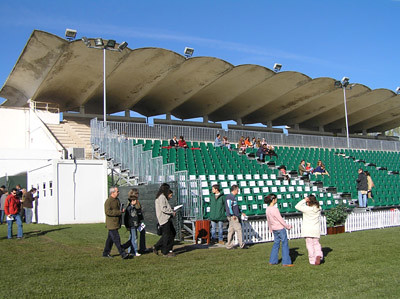On a bright, clear day with a vivid blue sky, the photograph captures a scene at an event held in a stadium, likely for a graduation or a basic sporting event. Prominent in the image are tall bleachers, predominantly green with some white rows towards the front, consisting of about 25 rows. The bleachers have an overhanging canopy supported by poles on either side, complete with spotlights above it. In front of the bleachers, a white picket fence can be seen, along with a grayish metal fence on the left side.

Several people are scattered around the grassy field in front of the bleachers, some facing various directions. They appear to be wearing casual clothing like jeans, jackets, and long-sleeved shirts, suggesting cooler weather. A few individuals are visible sitting in the middle and back of the bleachers, but most are standing or milling about. To the left of the bleachers, there is a white structure with doors and a few people near it. The atmosphere is bustling with people of various ages and races either sitting or arriving, holding pieces of paper as if for a ceremony.